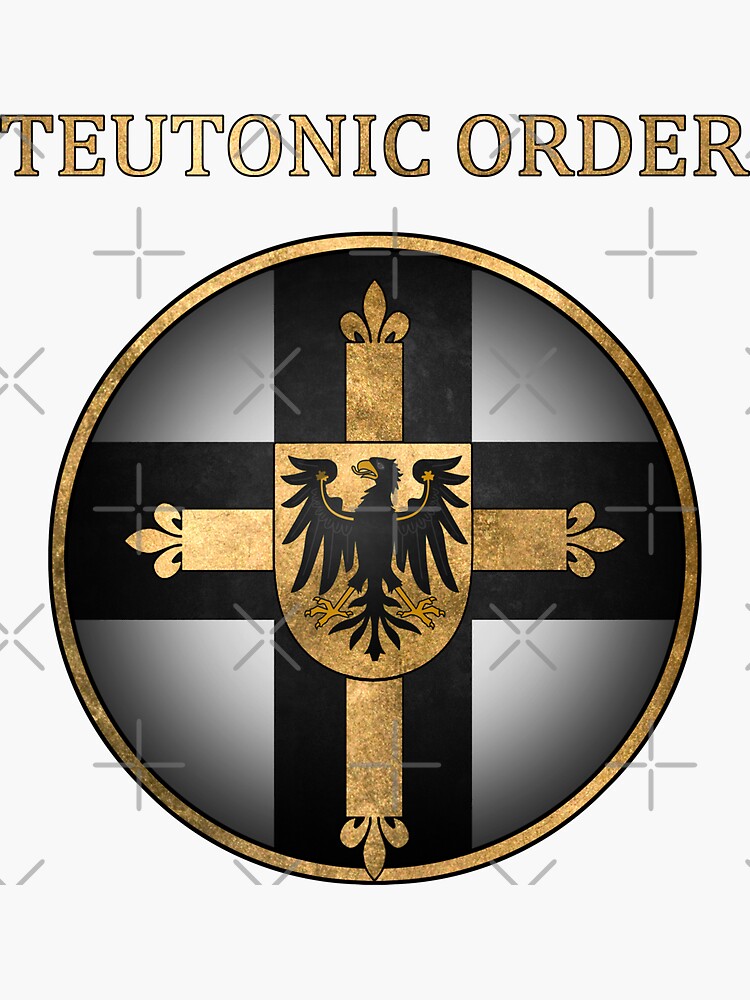This poster features a central circular crest on a white background. At the top, the bold gold and black-outlined text "Teutonic Order" is prominently displayed. The circular crest, which dominates the center of the poster, has a gold border outlined in black. Within this circle lies a large, thick black cross set against a gray background that fades to white towards the center. Positioned at the intersection of the black cross is a gold cross adorned with fleur-de-lis designs at each point. Nestled at the heart of the gold cross is a detailed coat of arms: a black bird of prey, perhaps an eagle or crow, with distinctive orange feet and beak. The bird, looking to the right, is portrayed with its tongue out and wings spread wide as if in a display of strength. Finally, in the bottom right corner, the small white text "Warlord Apparel" completes the image.